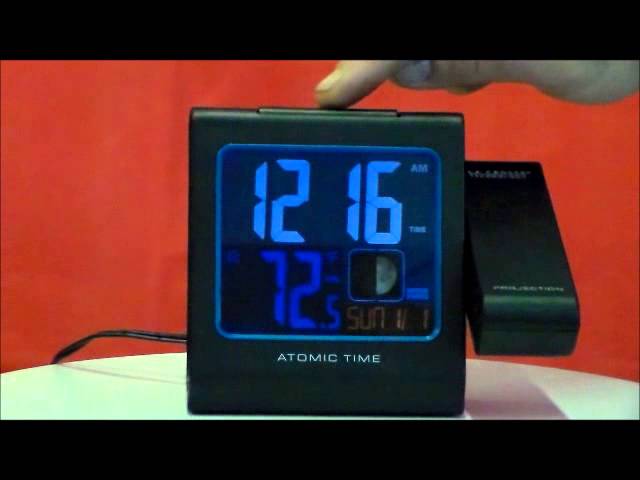In this photograph, a black square digital alarm clock with "Atomic Time" marked in white beneath its display rests on a white table. The time displayed is 12:16, with the digits illuminated in bright blue. Below the time, the clock shows smaller digits, reading 72.5 degrees, along with the day "Sunday" and the date "1". A small image of a half-covered moon is also visible on the clock's display. The clock features a large winding mechanism on its right side and an angled latch. A wire runs from the clock, presumably plugged into an unseen wall socket. The background is painted a vivid red. A single finger is gently pressing a button on top of the clock, captured just as it descends onto the button.